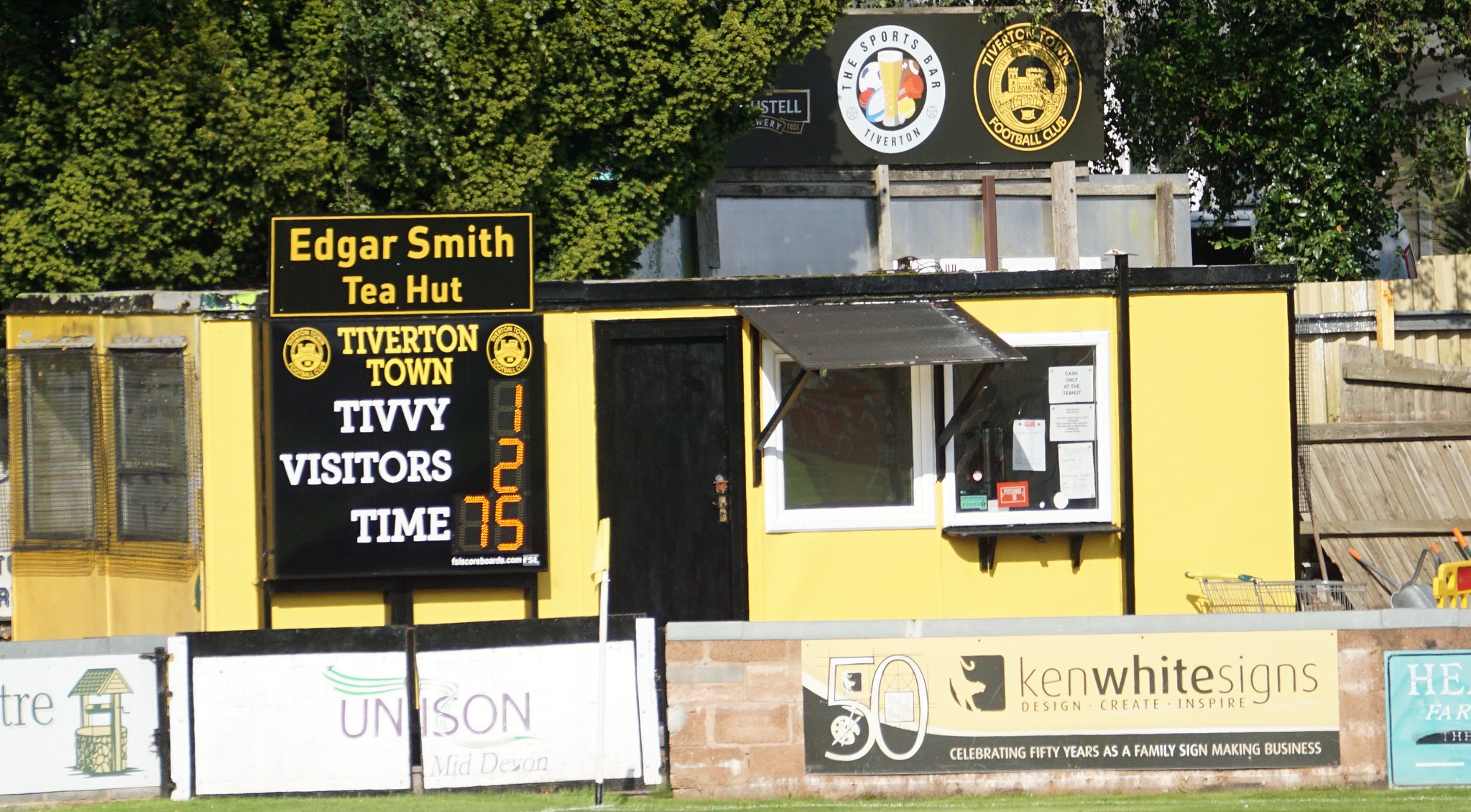In this daytime outdoor scene, we observe a modest yellow trailer-like building, known as the Edgar Smith Tee Hut, situated near a sports field and surrounded by lush green trees. The building features a central black door flanked by a window with a black metal awning. Above the window, which is plastered with notices, a sign in gold letters displays "Edgar Smith Tee Hut," and below it, "Tiverton Town." A scoreboard attached to the building shows "Tivvy 1 - Visitors 2" with 75 minutes remaining. Additional advertisements and logos adorn the structure, including one that reads "Unison" and another for "Ken White Signs." Nearby, a visible sign promotes the Tiverton Town Football Club and the sports bar, illustrated with images of various sports balls.